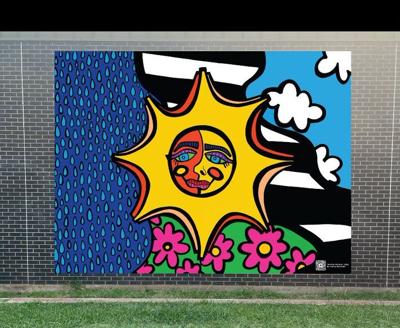The image depicts a mural that doesn't represent an actual scene but rather an artistic composition. The mural is framed with a gray brick wall that runs along both sides and a light green grass foreground. A black bar stretches across the top, occupying about an eighth of the image. The central focus is a cartoonish sun with a smiling face, blue eyes, and red lips, reminiscent of Native American art. This sun, set within a dark black circle and surrounded by yellow, banana-shaped rays, dominates the center of the mural. Below the sun, pink flowers with yellow centers dot the light green background. On the left side, dark blue and purple tones with turquoise raindrop-like designs descend vertically. The right side showcases a bright blue sky with whimsical, white, cartoon-style clouds. Additionally, a black and white pattern resembling piano keys loops around behind the sun, further adding to the mural's whimsical and eclectic nature.